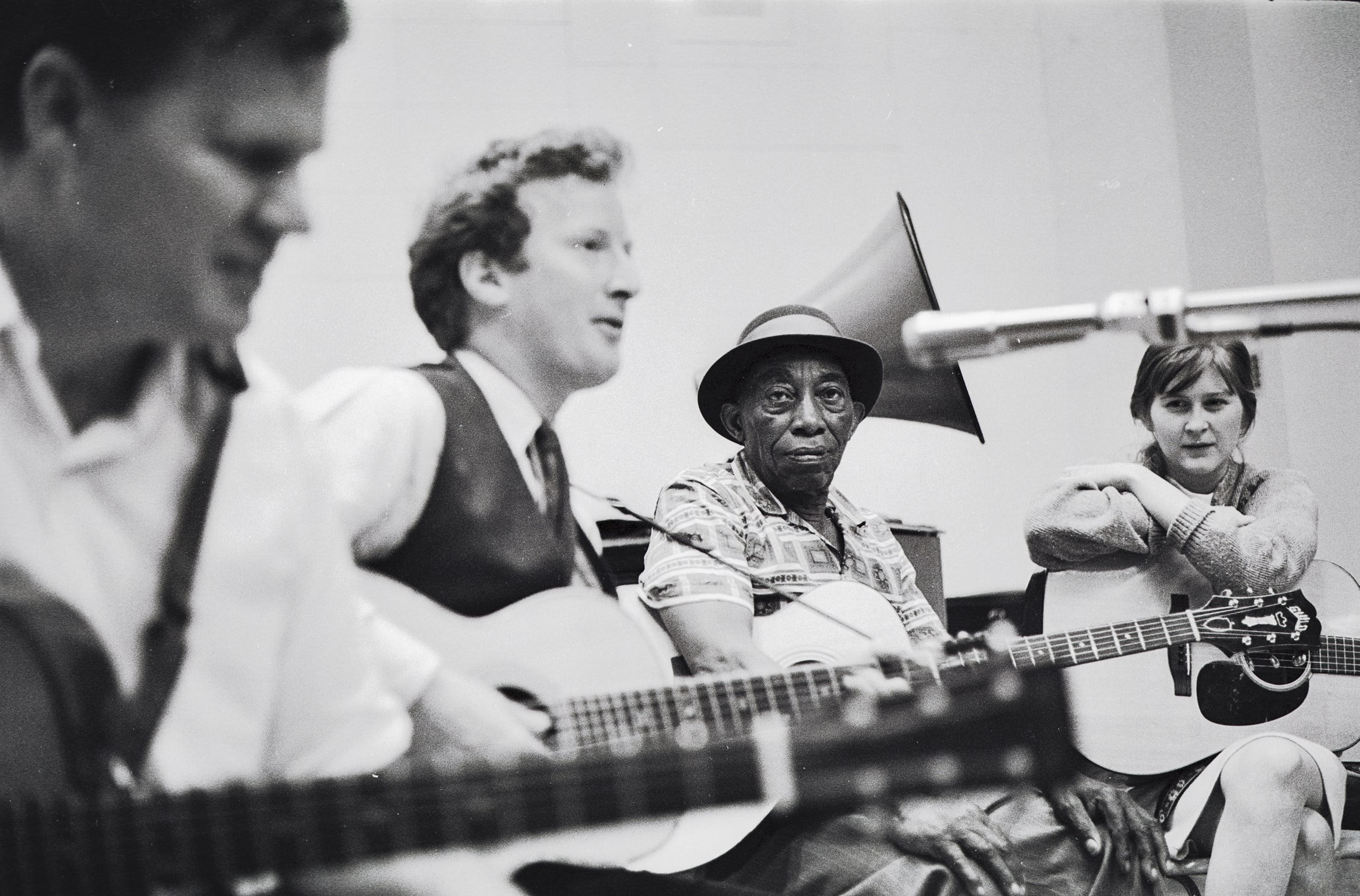A black-and-white image from potentially the 60s, 70s, or 80s captures a band of musicians seated with their acoustic guitars. Four people are in the shot, highlighting two white men on the left. One man, older with a patterned shirt and hat, gazes directly into the camera, his arm resting over his guitar. Beside him, a younger white man in a vest is focused on playing his guitar, strumming thoughtfully and looking off to the right. At the center, a black man wearing a bucket hat also stares into the camera, his arms around his guitar, with a vintage phonograph partially visible behind him. To the far right, a white woman with her arms resting atop her guitar, likely held at the elbow, also engages with the camera, distinguishing herself by not playing. The group is arranged around a central microphone, suggesting a performance or recording session.